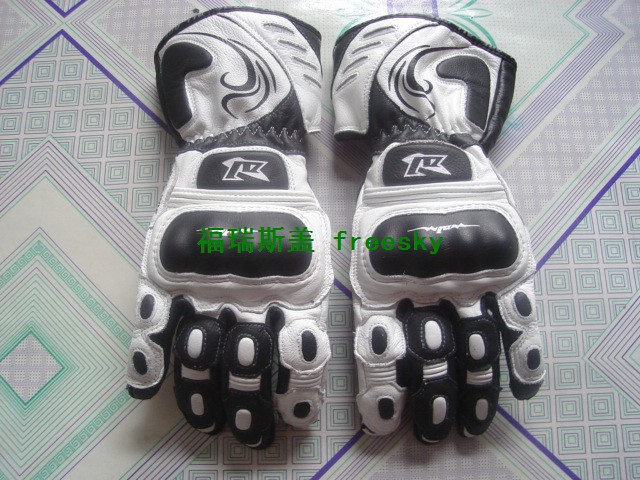This image features a pair of heavy-duty, technical sports gloves, predominantly black and white, designed for substantial activities possibly like ice hockey. The gloves are laid palm down against a background of pale, geometric-patterned tiles with teal, purple, and white hues, arranged diagonally. The gloves exhibit extensive padding and reinforcement, especially over the knuckles and finger joints. The main body of the gloves is white, adorned with intricate black inlays. Notably, the pinky and forefinger of each glove are white with black dots, while the middle and ring fingers are black with white dots. The knuckles have black-padded reinforcements, and there's a plastic-looking area protecting them. Near the wrist, a small black rectangle houses a barely visible logo consisting of squiggly black and white letters. Additionally, the wrist portion features a loose white cloth section embellished with paisley-esque black swirls, extending slightly onto the forearm for added protection. The top of the glove also displays an emblem resembling a white triangle with elements that look like a basketball hoop, including elaborate green Chinese characters alongside the word "FREESKY," likely denoting the brand name.